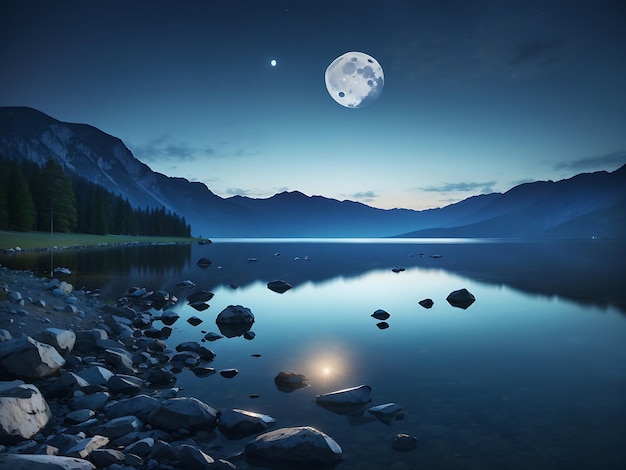The image showcases a serene, possibly computer-generated portrayal of a mountainous lake at night, with a slightly cartoonish feel. Dominating the sky is a very large full moon, accompanied by a single star to its left. The moonlight reflects beautifully off the clear, glassy water of the lake, which is edged and interspersed with craggy, jutting rocks. Majestic mountains frame the scene, with tall pine trees lining the shores and extending into the mountainous terrain. The atmosphere feels clean and tranquil, though somewhat surreal. As the sun has recently set, a vibrant blue sky transitions into night, enhancing the peaceful ambiance of this idyllic mountain landscape.